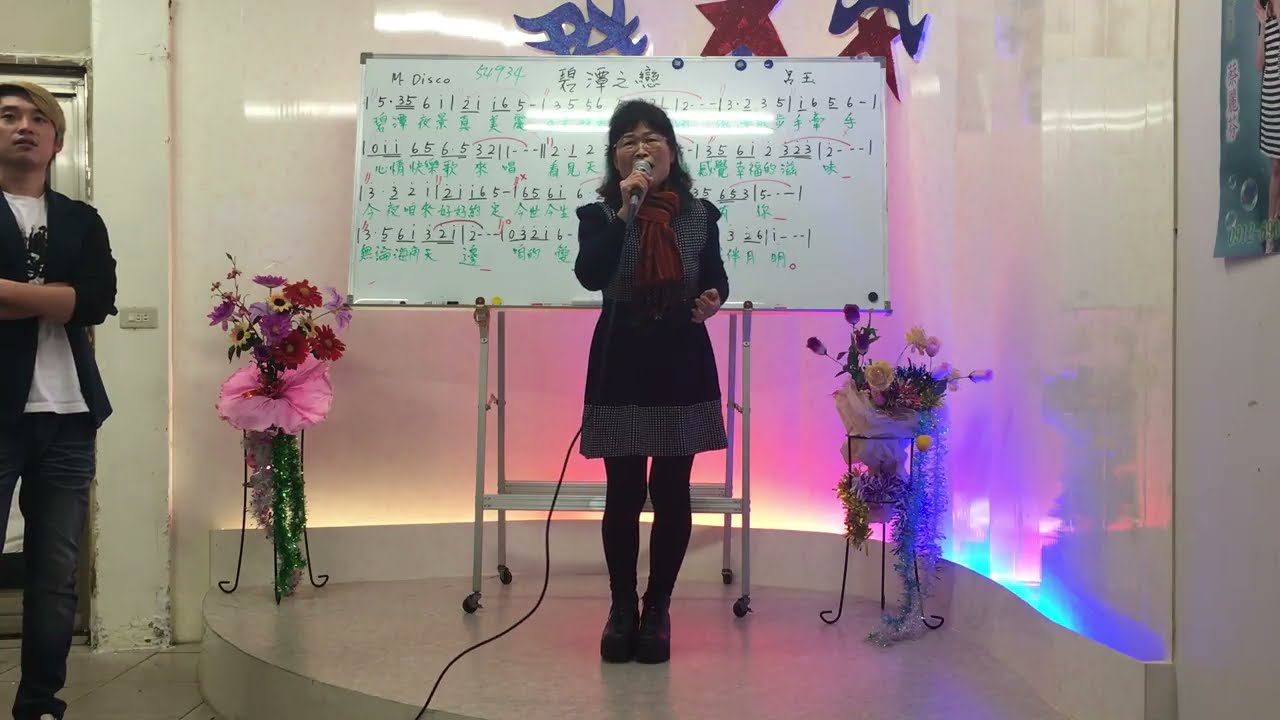An older Asian woman with black shoulder-length hair and glasses stands on a small, white, raised, rounded stage. She is holding a wired microphone close to her open mouth, appearing to sing or announce something. She is dressed in a blue long sleeve dress paired with black tights, black shoes, and a tied burgundy scarf. Her attire also includes a black vest. Behind her, a large whiteboard displays numbers and various Asian characters, likely Chinese or Japanese. Reflective, colored lights bounce off the stage backdrop, illuminating it in shades of blue, red, pink, white, and yellow. Flanking the whiteboard are decorative planters filled with floral arrangements. To the left side of the stage, an Asian man with blonde hair, wearing a white t-shirt under a black sweater and dark pants, stands observing the scene.